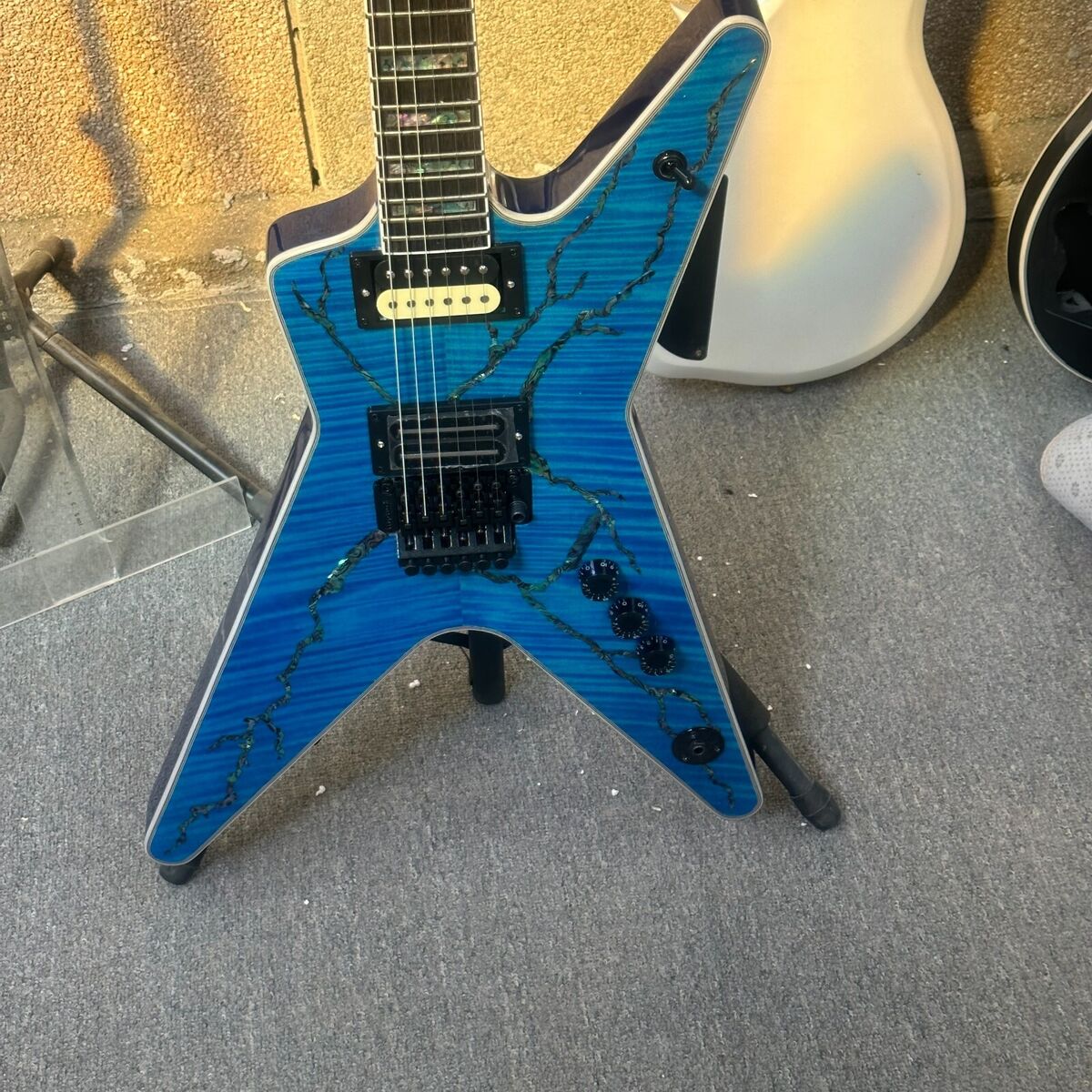This color photograph, captured in natural sunlight, depicts an electric guitar with a distinctive, star-like or lightning bolt shape. The guitar features a deep blue base color, accented by lighter blue stripes and jagged black lines resembling lightning streaks splintering across its front. The lines appear slightly sparkly, adding a textured, shimmering effect. The guitar stands upright on a black stand against what appears to be a gray carpeted floor, with one leg of the stand visible. The background includes a concrete or brick wall reflecting yellowish sunlight, contributing to the outdoor feel of the image. Behind the focal guitar, you can see the body of a plain white guitar standing against the wall, with a tiny portion of a black electric guitar peeking out from the right side. To the left side of the photograph, part of an acrylic music stand is also visible.